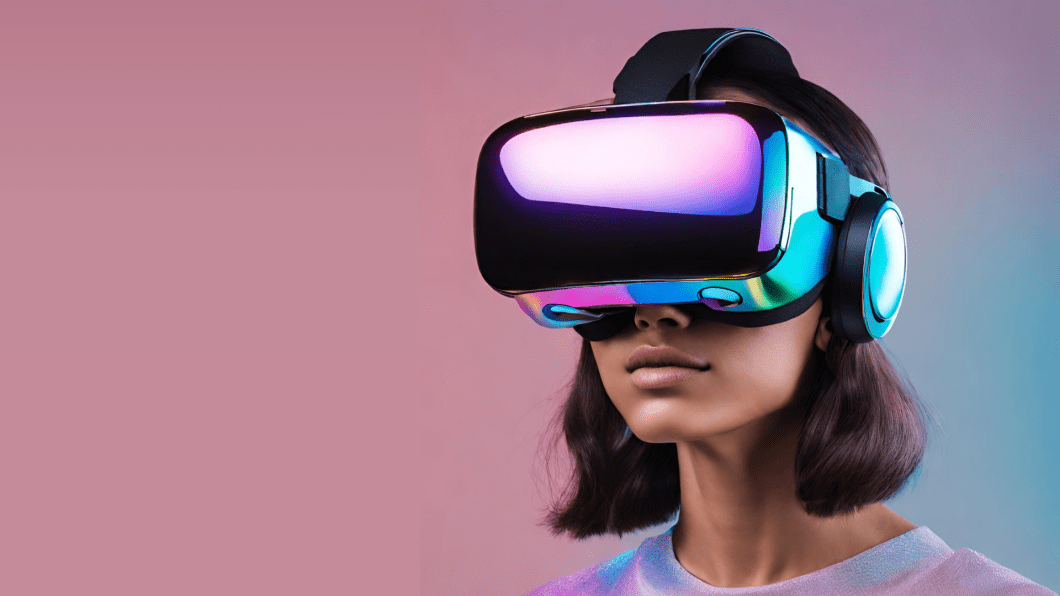This photograph features a young girl, likely a teenager, wearing a cutting-edge virtual reality headset. The VR headset is predominantly metallic blue with reflective, shiny black lenses, and exhibits gradient shades of purple, green, and blue around the lens and earphones. The headset straps go around her ears and over the back of her head, securing it firmly in place.

The girl has dark hair that falls slightly past her shoulders and she is captured in a three-quarters view, looking intently into the VR headset. She appears to be engrossed in an immersive three-dimensional picture being projected into the goggles. 

Her attire—a shirt that appears to be either tie-dyed or affected by the ambient lighting—features hues matching the headset's color scheme, including streaks of blue, pink, rose, lavender, and pale blue. The backdrop starts with a light blue or greenish-blue hue and transitions gracefully into a pinkish or mauve shade, providing a visually cohesive and immersive scene that complements the futuristic vibe of the VR experience.